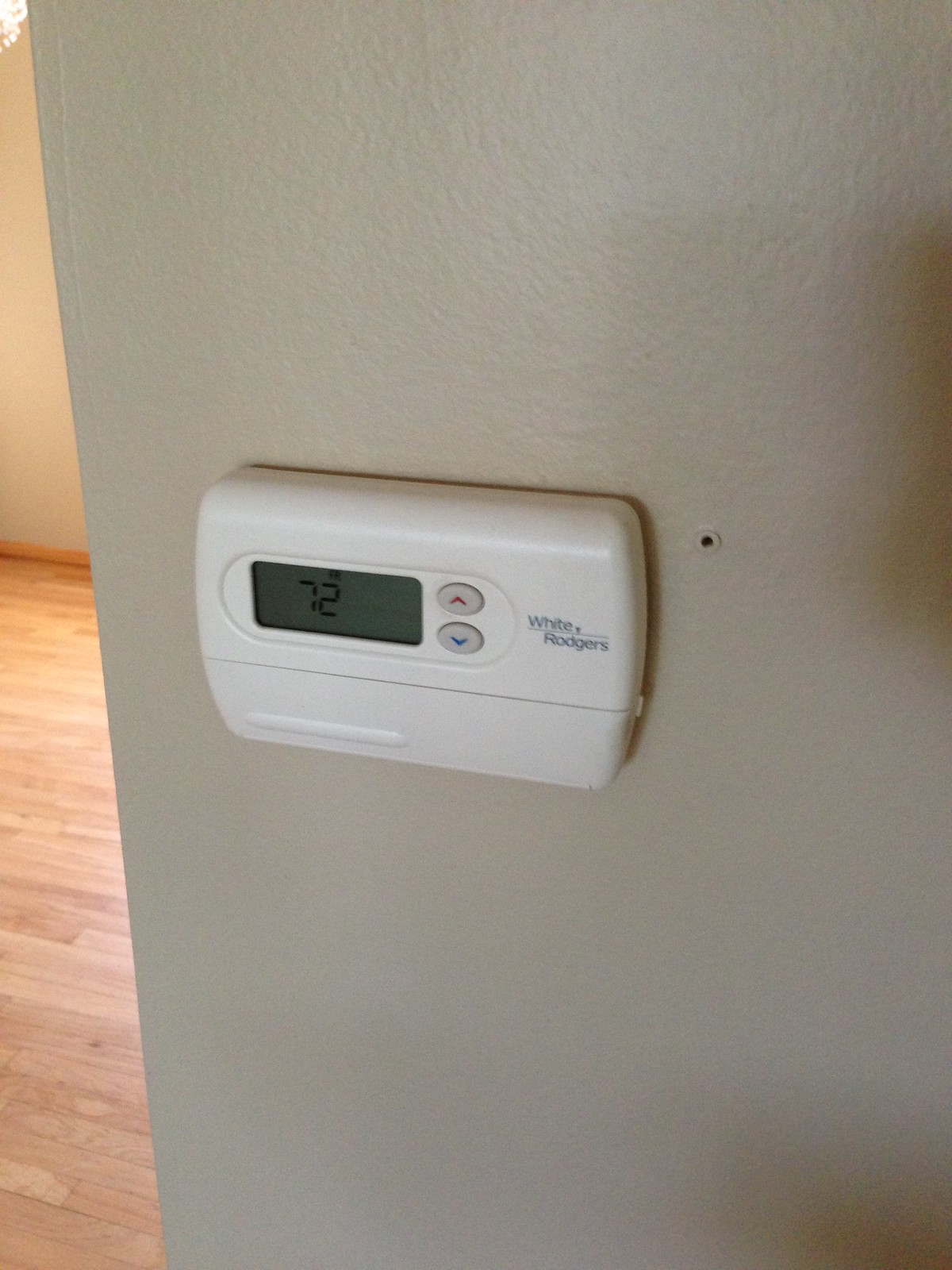The photograph showcases a thermostat mounted on a beige-painted sheetrock wall, characterized by its smooth surface with a slight orange peel texture and a semi-gloss finish. The beige wall contrasts subtly with the creamy white plastic of the thermostat, which prominently displays the brand name "White and Rogers." The thermostat features a clear digital display indicating a temperature of 72 degrees, flanked by two buttons - a red one for increasing the temperature and a blue one for decreasing it. A small graspable lip on one side suggests it can be opened for additional controls or programming. Just to the right of the thermostat is a tiny, deliberate hole, likely for mounting purposes. The image captures a shadow cast by the thermostat onto the wall, hinting at the presence of the person taking the photo. To the left, part of the room becomes visible, revealing a hardwood floor and another cream-colored wall bathed in daylight, adding a sense of depth and context to the scene.